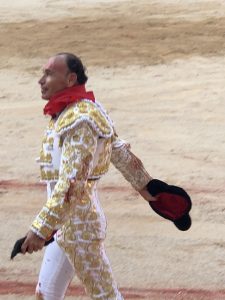The photograph captures a Hispanic male, presumably a Spanish bullfighter, standing in an outdoor arena with a dirt floor. He is dressed in traditional bullfighting attire, characterized by a striking white outfit adorned with intricate gold designs that decorate his shoulders, arms, and chest. A vivid red scarf is neatly tied around his neck, adding a pop of color. In his right hand, extended slightly backwards, he holds a black hat, while his left hand grasps a black piece of fabric. His hair is short and noticeably receding at the hairline. The background of the image showcases a sandy, light to dark brown arena floor, typical of a bullfighting setting.